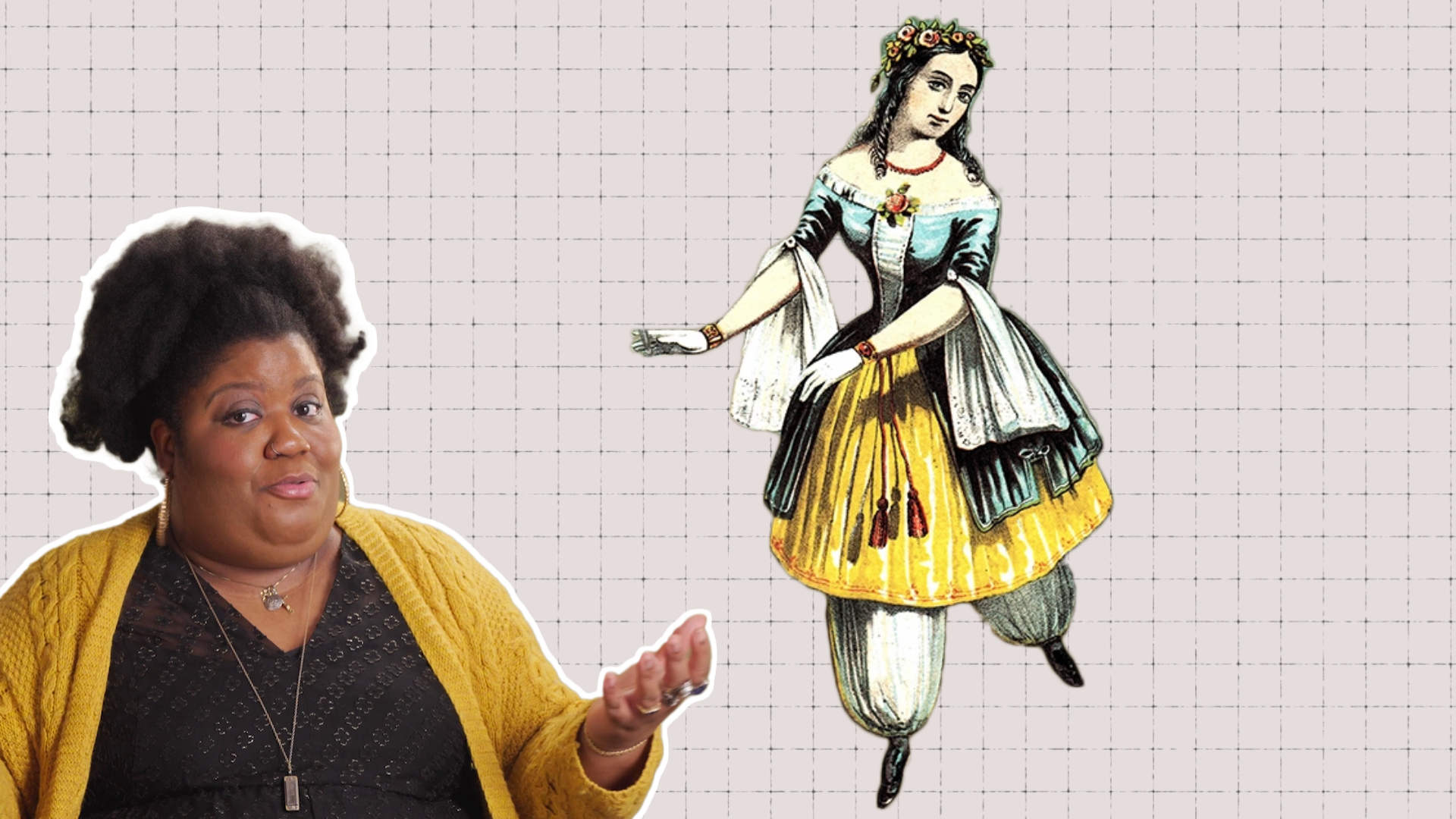This is a wide rectangular digital artwork featuring a background reminiscent of graph paper, with light off-white coloring and thin gray grid lines. Just to the right of the center, there is a cutout of a color drawing of a woman dressed in an off-the-shoulder blue lacy top paired with a wide yellow skirt adorned with white stripes. She complements this outfit with billowy white pantaloons and thin black ballet slippers. Her long black hair is decorated with flowers, and she wears white gloves, with her arms positioned towards the left side as if in dance. In the bottom left corner, there is another cutout, bordered slightly in white, depicting a black woman. She has her hair neatly pulled up and wears a silver pendant necklace over a black V-neck shirt, topped with a yellow cable knit sweater. Her expression suggests she is either explaining something or asking a question, indicated by her outstretched arm and engaged demeanor.